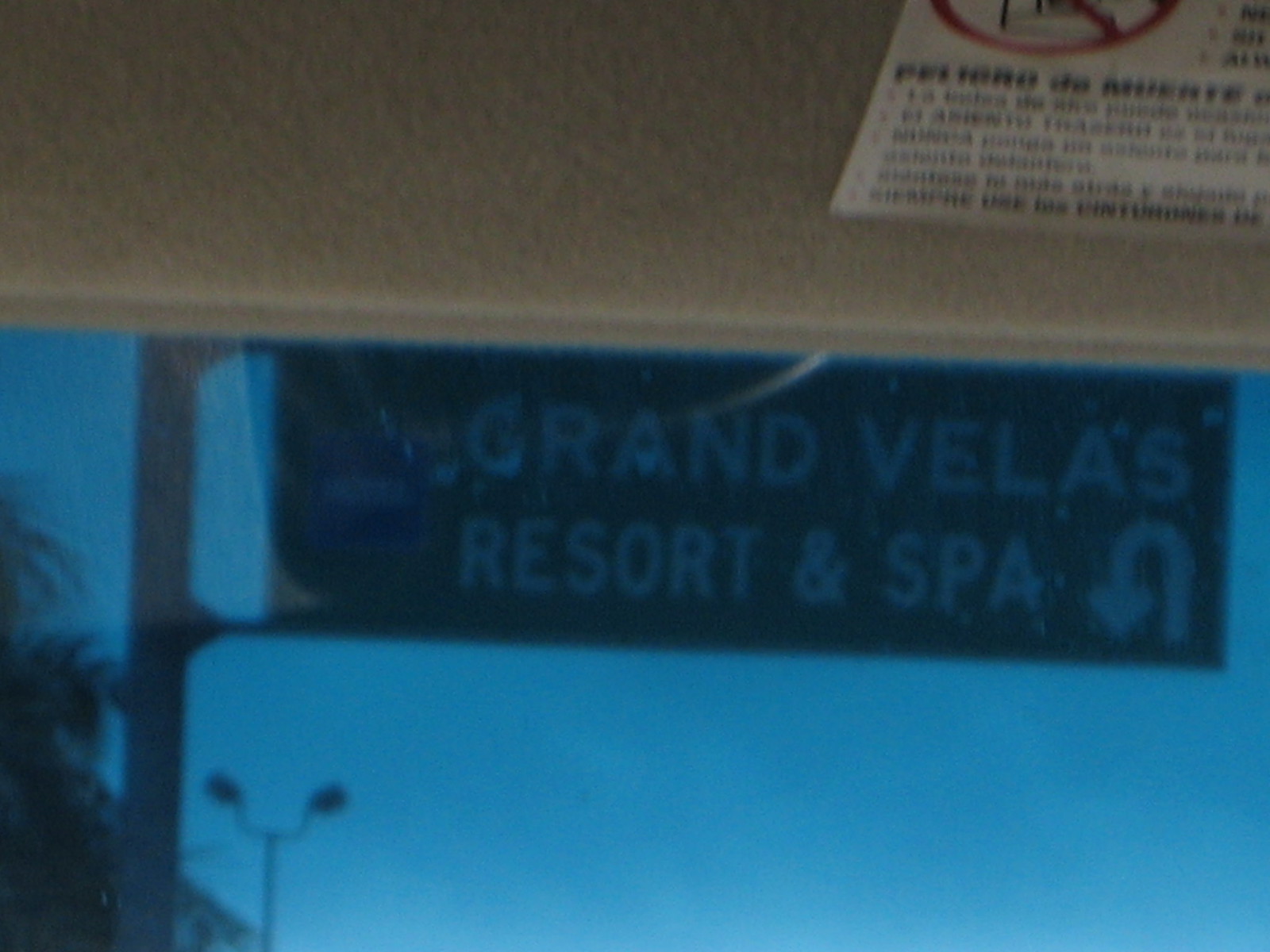A low-quality color photograph, likely taken from inside a car through the windshield, captures a scene from either the driver's or passenger's side. The top portion of the image is dominated by the underside of a sun visor, featuring a black-text warning label in the top right corner. Dominating the middle section of the photo is a large street sign announcing "Grand Velas Resort and Spa" with a U-turn arrow, set against a backdrop of a dark, possibly twilight sky. The sky's deep blue hue suggests either early morning or late evening. In the lower left quadrant, a street lamp with twin lights is visible, along with the hint of a tree, adding elements of urban and natural scenery to the composition.